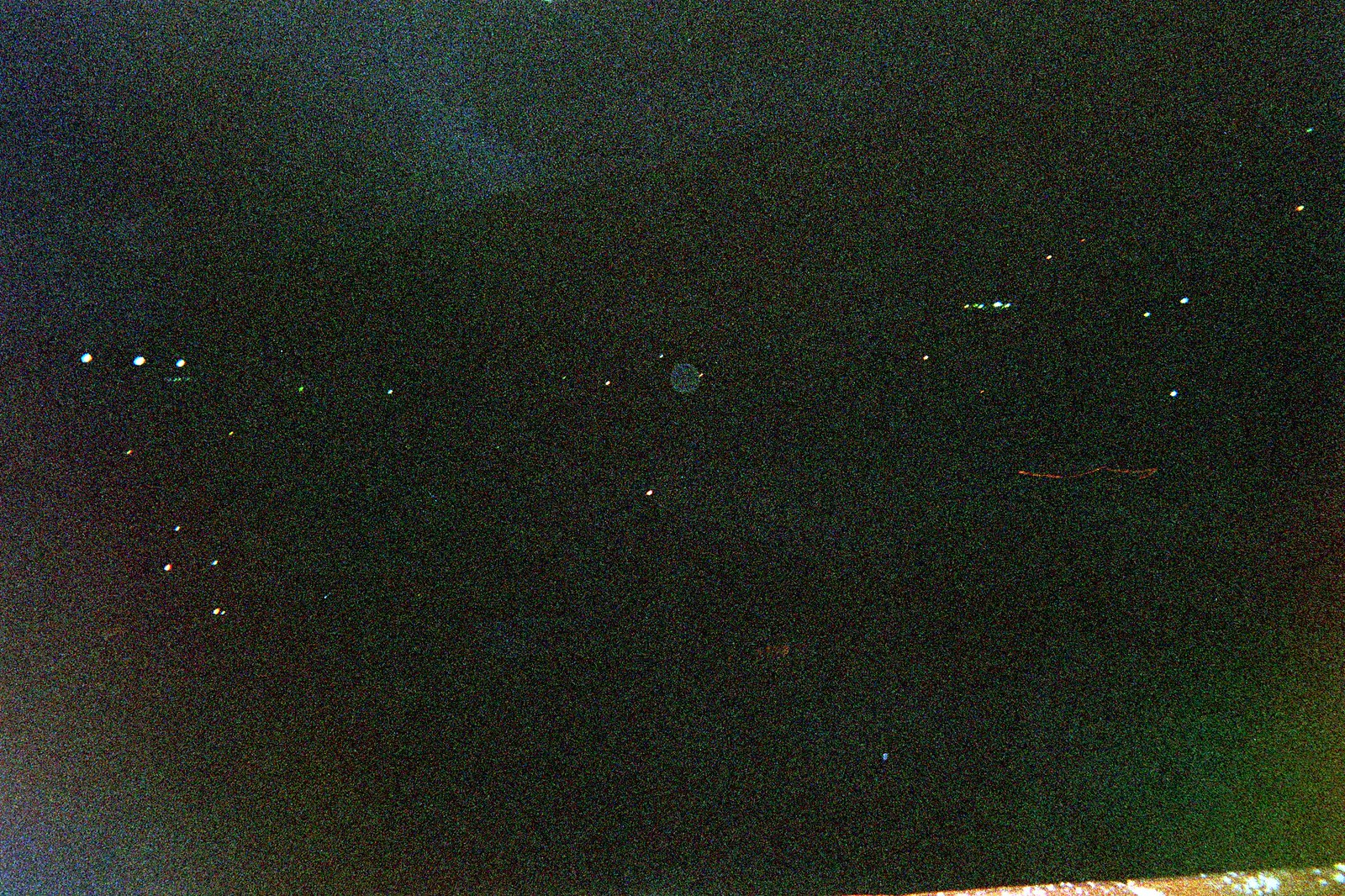This rectangular landscape image, approximately 50% wider than it is tall, predominantly features a dark gray to nearly black background with a distinct, chalky or grainy texture. Occupying about 95% of the image, this dark expanse is only interrupted by a small, rusted brown railing in the bottom right corner, which runs horizontally and barely intrudes into the frame.

Scattered throughout the dark, textured background are an array of lights. These lights vary slightly in size, with most appearing as pinpoints or slightly larger dots. In the upper left portion of the image, three lights are aligned horizontally, standing out a bit more prominently. While some of the lights could be mistaken for distant stars, they generally resemble artificial lights seen from afar. Despite the presence of these lights, the image largely retains its dark and grainy character.